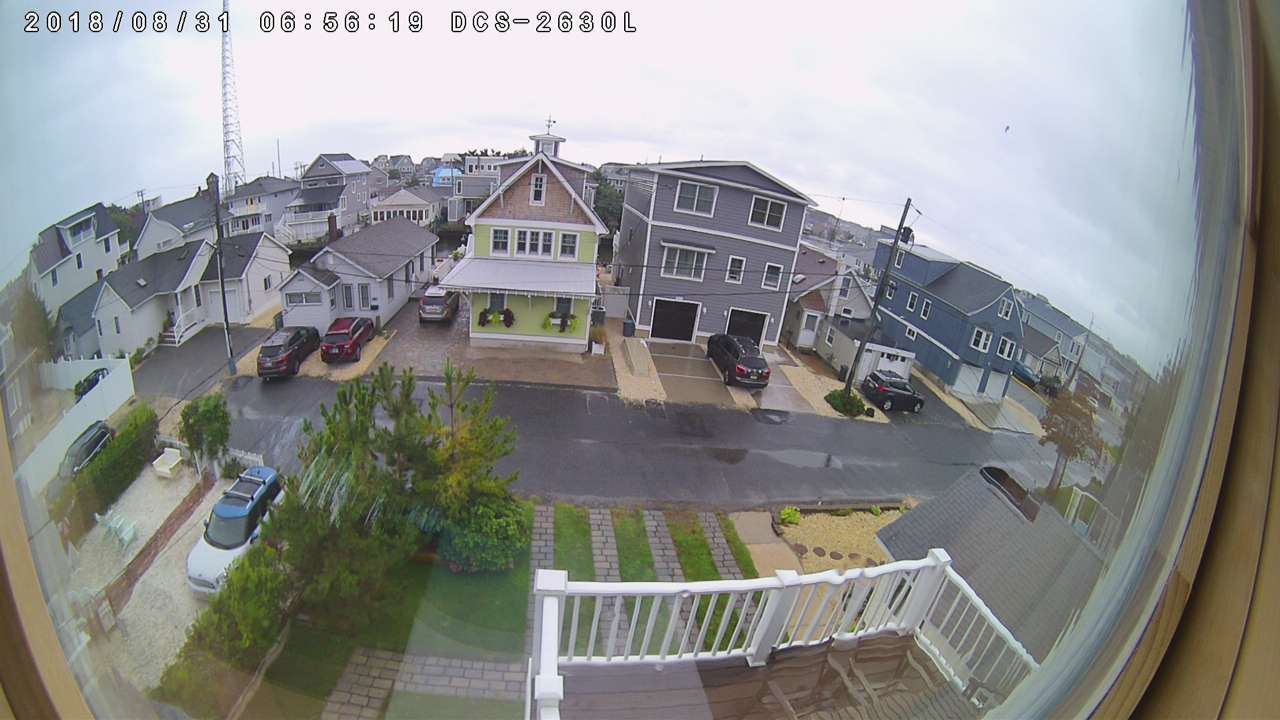This photograph, seemingly captured from an upstairs window of a residential home on August 31st, 2018, at 6:56 AM, provides a detailed view of the front yard and the surrounding neighborhood. The camera overlooks a brick walkway in the front yard, flanked by lush trees and bushes. To the left, a car is parked in the driveway, while on the right, the roof of a neighboring house is visible. A balcony from the upper level can also be seen. The street, running horizontally through the middle of the photograph, separates the observed property from a row of homes on the other side. Prominently, a lime green painted house stands at the center, bordered by a large gray house to its right and a blue house further right. The sky overhead is a serene blue, adorned with wispy white clouds, adding to the tranquil suburban scene. The neighborhood appears to consist of primarily two to three-story homes, some with garage levels and others with small individual features, creating a cohesive yet varied residential landscape.